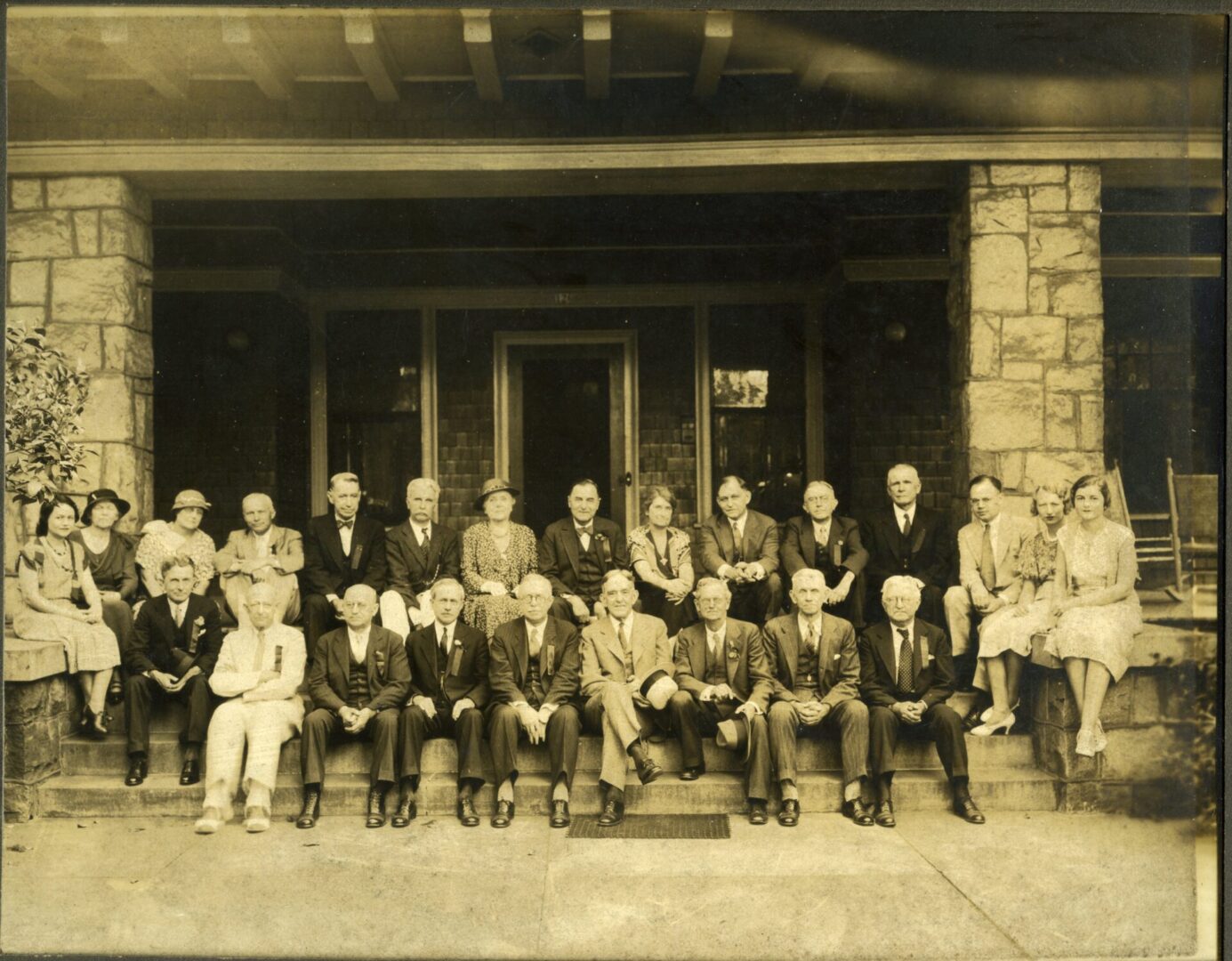This is a wide shot of a vintage black and white photograph, possibly taken in the 1940s or 1950s, featuring around 25 people gathered on the front steps of what appears to be an old lodge or club. The photo shows signs of aging, with a yellowed tint. The group consists mostly of older men and a few women, both young and old. The men, many with gray hair and balding, are dressed in suits and ties, while the women wear skirts, dresses, and high heels. They are all posing for the camera, with some men smiling and others frowning. The people are seated on the wide concrete stairs leading up to a house or building with distinctive architectural features, including slate pillars made of white large block stone and a wooden roof covering the porch area. The entrance features glass doors with bricks above them. The setting includes a driveway of white concrete in front of the steps. The image captures a formal and nostalgic moment, with everyone dressed in the elegant clothing styles of the mid-20th century.